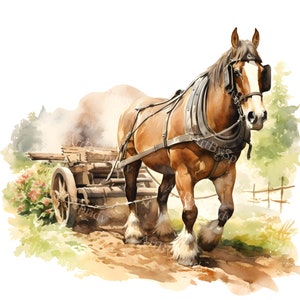This detailed watercolor painting depicts a powerful, brown Clydesdale-type horse adorned with leather blinders and a white streak down its nose, pulling an old-fashioned wooden cart filled with stacked wood. The horse's muscular physique is highlighted, along with its fluffy white fur around each hoof. It wears a dark brown leather yoke and reins that attach it to the cart. The scene is set on a dirt road, flanked by greenery and colorful flowers, with a fence line and mountains in the background under swirling skies. The irregular edges of the painting contribute to its rustic charm.